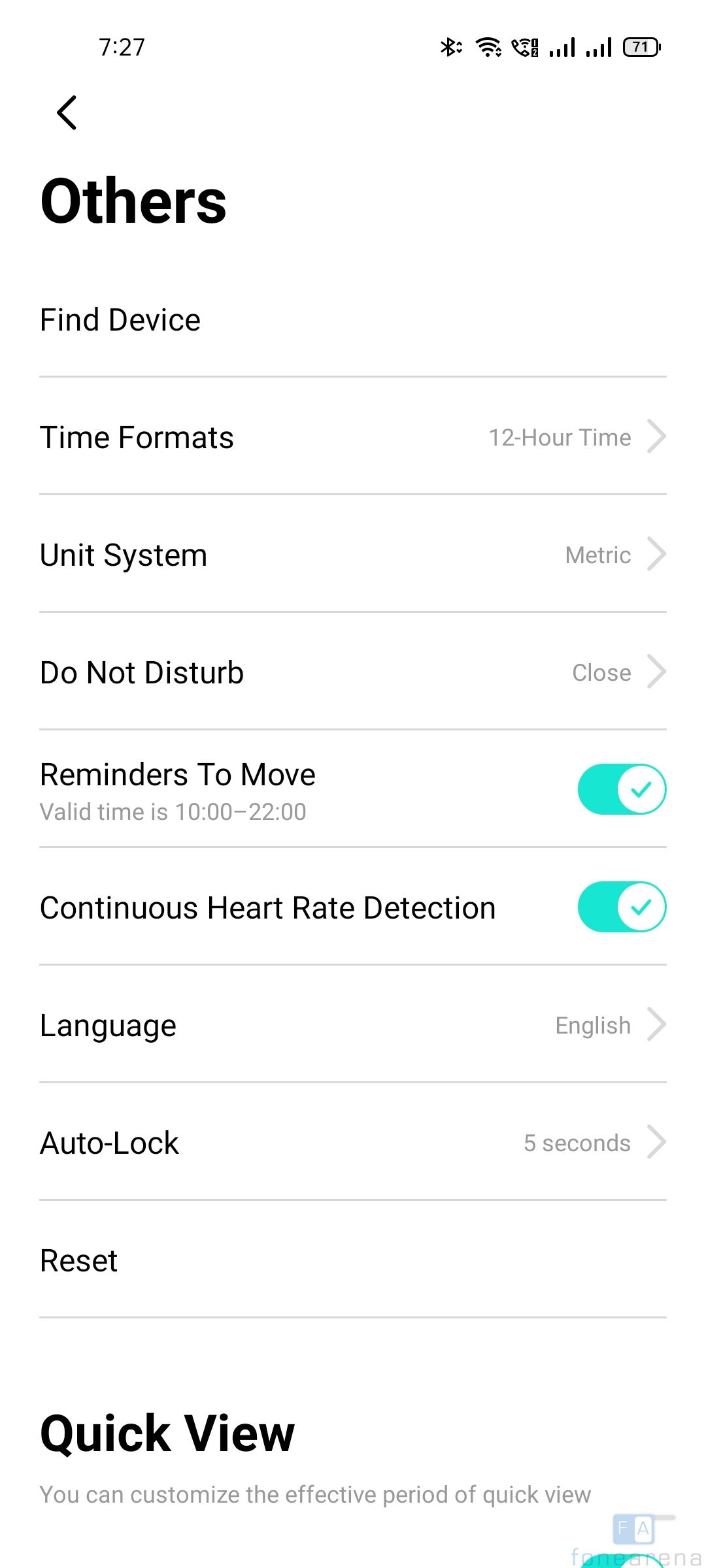The image is a screenshot of a cell phone screen taken at 7:27 AM, as indicated by the time shown in the upper left-hand corner. On the upper right-hand side, there are multiple icons: a battery icon displaying '71,' two cellular signal indicators, Wi-Fi signal, and a Bluetooth signal. An unknown icon is situated between the Wi-Fi and cellular signal indicators.

In the upper left corner, an arrow pointing to the left is labeled "Others" in bold black font. The background of the screen is entirely white, creating a clean appearance. The screen displays several settings: 

- "Find devices"
- "Time format," which is set to the 12-hour format
- "Unit system," set to metric
- "Do not disturb," which is currently turned off
- "Reminders to move," active between 10:00 and 22:00 with a green highlight and check mark
- "Continuous heart rate detection," also highlighted in green with a green check mark
- "Language," set to English with an arrow for more options
- "Auto lock," set to 5 seconds
- "Reset"

At the very bottom, the screen shows "Quick view" in bold black letters, followed by a note that reads, "You can customize the effective period of quick view."